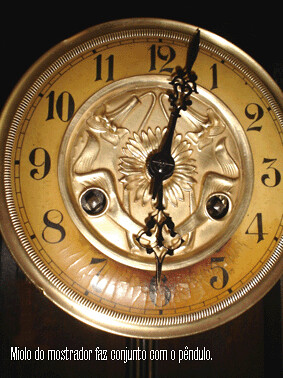This vibrant color photograph showcases a close-up of an ornate, round clock face against a black background. The clock's golden rim, which is illuminated at both the top and bottom, frames almost the entire face, with only the very left and right edges slightly cropped out of the shot. The clock face itself is a deeper gold, adorned with numbers ranging from 1 to 12, and is encircled by a black inner ring featuring intricate embossing that catches the light, giving it a lighter appearance than its outer gold rim.

Within this inner black circle are two smaller circles toward the bottom and another centrally located circle, adding to the detailed craftsmanship of the clock. The clock's hands are elaborately decorated in black; the long minute hand is positioned between 12 and 1, featuring a decorative element near its tip, while the shorter hour hand points towards the 6. At the bottom of the clock face, there is some slightly blurred white text, which appears to be in a language other than English, adding an element of mystery and intrigue to the elegant timepiece.